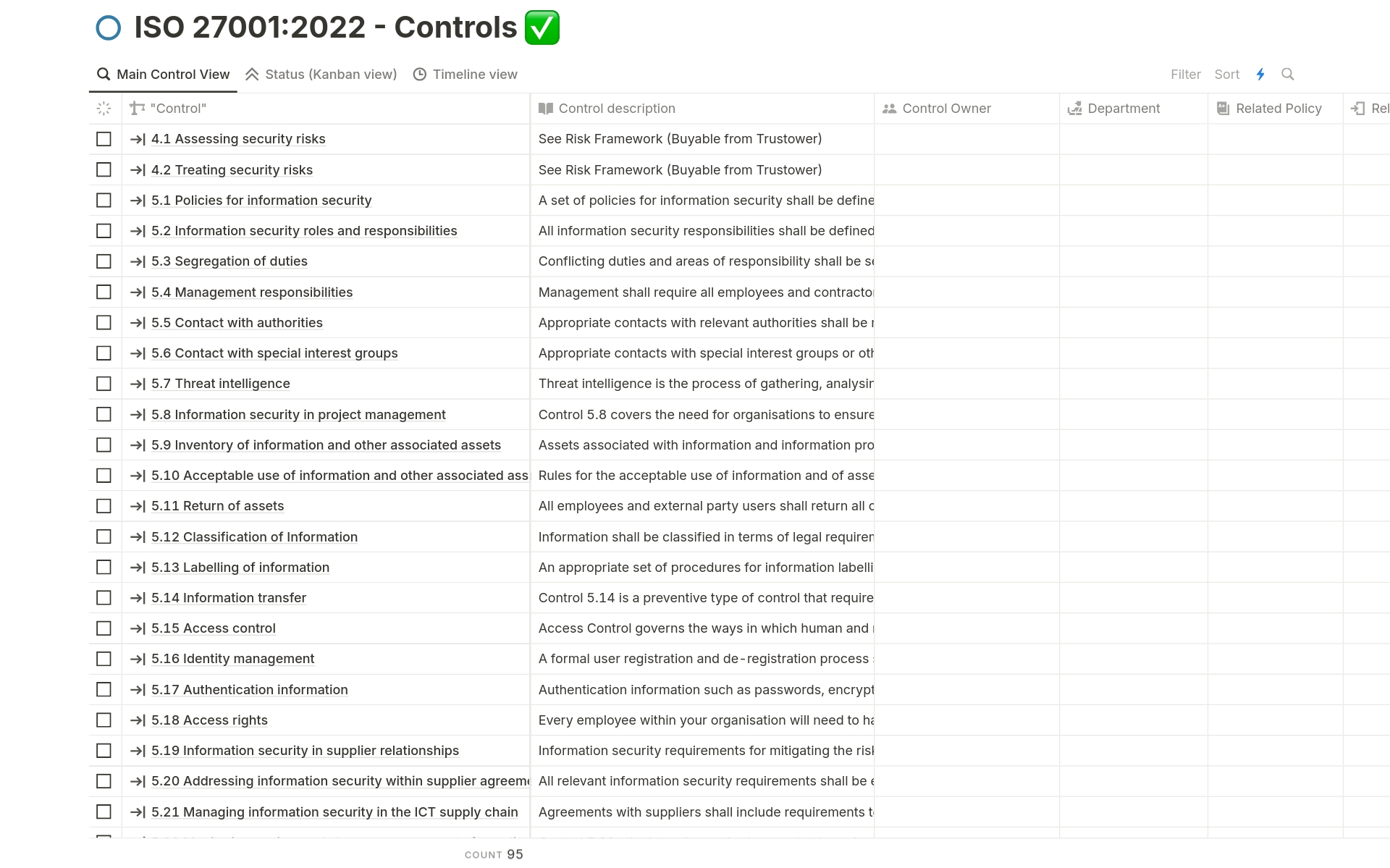The image shows a detailed printout that appears to be a screen capture of a dashboard or a document related to ISO 27001:2022 controls. In the top left corner, there is a title "ISO 27001:2022 - Controls" accompanied by a green box with a white checkmark inside. Below this, the layout resembles an Excel spreadsheet with multiple columns and rows.

In the first row, the columns are labeled as follows: "Hourglass", "Main Control View", "Status", "Kanban View", and "Timeline View." This suggests different ways to view or filter the information.

Below these headers, various control titles are listed down the rows in their respective columns. For instance:

1. **Assessing Security Risks**: The description states, "See risk framework viable from Trust Tower."
2. **Treating Security Risks**: Similarly, it also mentions, "See risk framework viable from Trust Tower."
3. **Policies for Information Security**: This entry notes that "A set of policies for information security shall be defined."
4. **Information Security Roles and Responsibilities**: The description specifies that "All information security responsibilities shall be defined."
5. **Segregation of Duties**: The description discusses that "Conflicting duties and areas of responsibility shall be managed."

Further down the list, it includes:
6. **Management Responsibilities**: It is detailed that "Management shall require all employees and contractors to adhere to specified guidelines."

The printout goes into more detail about these controls, their statuses, and descriptions of the requirements, staying consistent with the structured format typically seen in compliance documentation.

Overall, this image is a rich, visually ordered summary of various ISO 27001:2022 controls, displaying their titles, descriptions, and statuses in a highly organized manner.